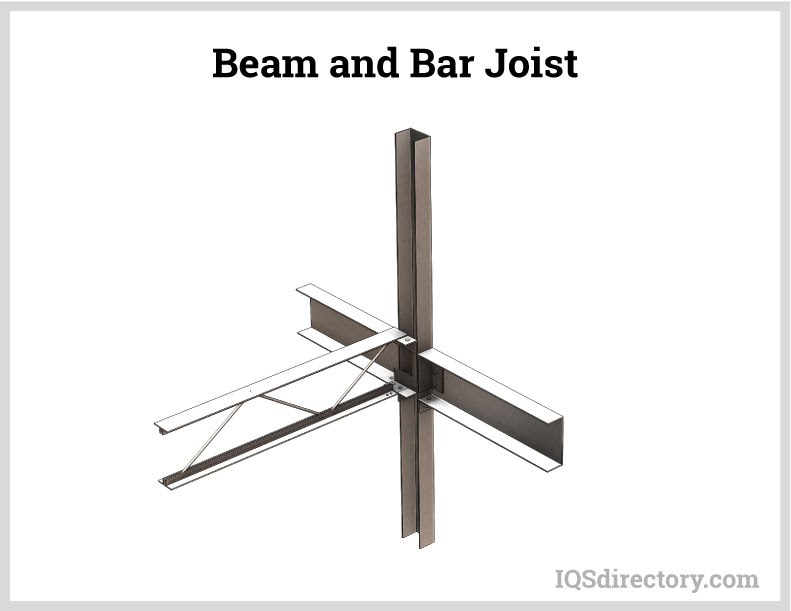This large square image features a thick gray border and a solid white background. At the top center, black text reads "BEAM and BAR JOIST," with capital letters for "B," "B," and "J," and the rest in lowercase. In the lower right-hand corner, gray text says "iqsdirectory.com." Central to the image is a detailed, drawn depiction of a metal beam and bar joist, appearing in a brownish color with white highlights. The primary vertical beam is crossed by a wider horizontal beam, which has dark gray flat parts and white-lipped edges. Another horizontal bar extends perpendicularly from this beam, connected by smaller zigzagged bars creating a support structure. This image illustrates a metal support system likely used in construction for flooring in buildings such as houses or offices.